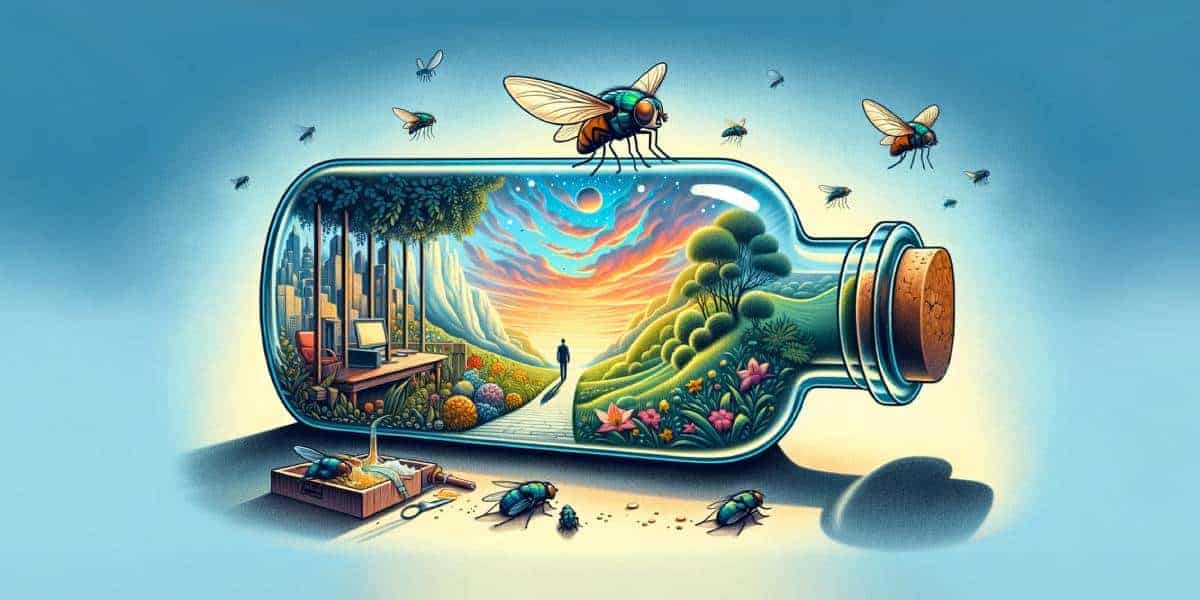This illustration depicts a fantastical scene contained within a shiny glass bottle, lying on its side and sealed with a cork. Surrounding the bottle, several flies of various colors, including blue, orange, and yellow, are flying around, with one perched on top and a few notably large flies in the foreground. Inside the bottle, there's a vibrant, saturated world featuring a pathway that runs through the center, bordered by whimsical trees and flowers. To the left, a cityscape with tall buildings emerges, while nearby, a computer desk is oddly integrated into the hillside. Above, a swirling sunset or sunrise mingles with clouds and celestial bodies like the moon and planets. This surreal, densely detailed miniature landscape juxtaposes urban, natural, and fantasy elements, all beautifully captured within the glass confines of the bottle.